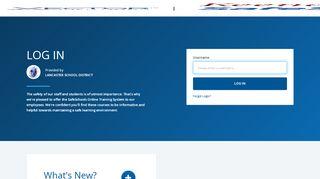The image depicts a small, somewhat pixelated interface, likely from a digital platform. At the top of the image, there's a light greyish panel featuring a compressed logo on the right-hand side, which appears to contain brown and blue hues, though the design is indistinct. The background beneath this panel is predominantly blue. On the left-hand side, large capital letters spell out "LOGIN." Below this heading, a circular icon, possibly illustrating a human head, is visible. Further down, a paragraph of white text is present, positioned underneath the login button. 

To the right of the "LOGIN" text, a white floating panel appears, presumably the login dialog. This panel includes an edit field for entering either a username or an email address. Beneath the field, there's a blue button labeled "LOGIN" in white font, although the text is very small and difficult to discern. In the bottom-left corner of this login dialog, additional text is visible, but its content is unclear.

Below the blue background, there's another greyish panel. This section features a cropped image displaying the partial text "WHATSNEW?", with the rest of the content obscured by the crop.